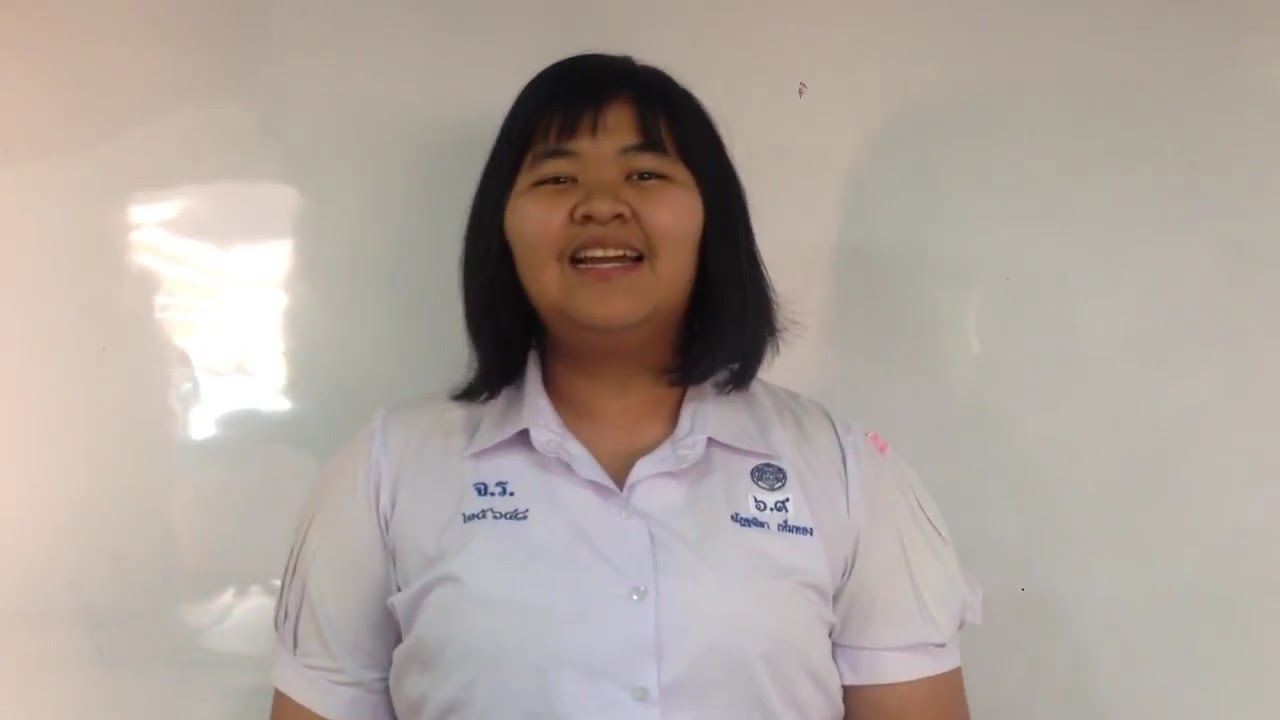The image features a young Asian woman with a round face and shoulder-length black hair, smiling warmly as she looks directly into the camera. She is wearing a white short-sleeved work uniform with a button-down front and a white collar, which gives the impression that she could be medical personnel, possibly a nurse or a health worker. On the left side of her uniform, there is an insignia that reads "DJ" with additional text beneath it that is not fully legible, suggesting her name. On the right side of the uniform, there is another emblem that includes a trademark and text resembling "B.GT," accompanied by what appears to be an image of a pizza. The background is a solid white wall, contributing to the crisp and clean setting, although there is a bright area on the left side of the image, possibly due to light reflection. Shadows from the lighting are visible around her head, enhancing the three-dimensionality of the scene.